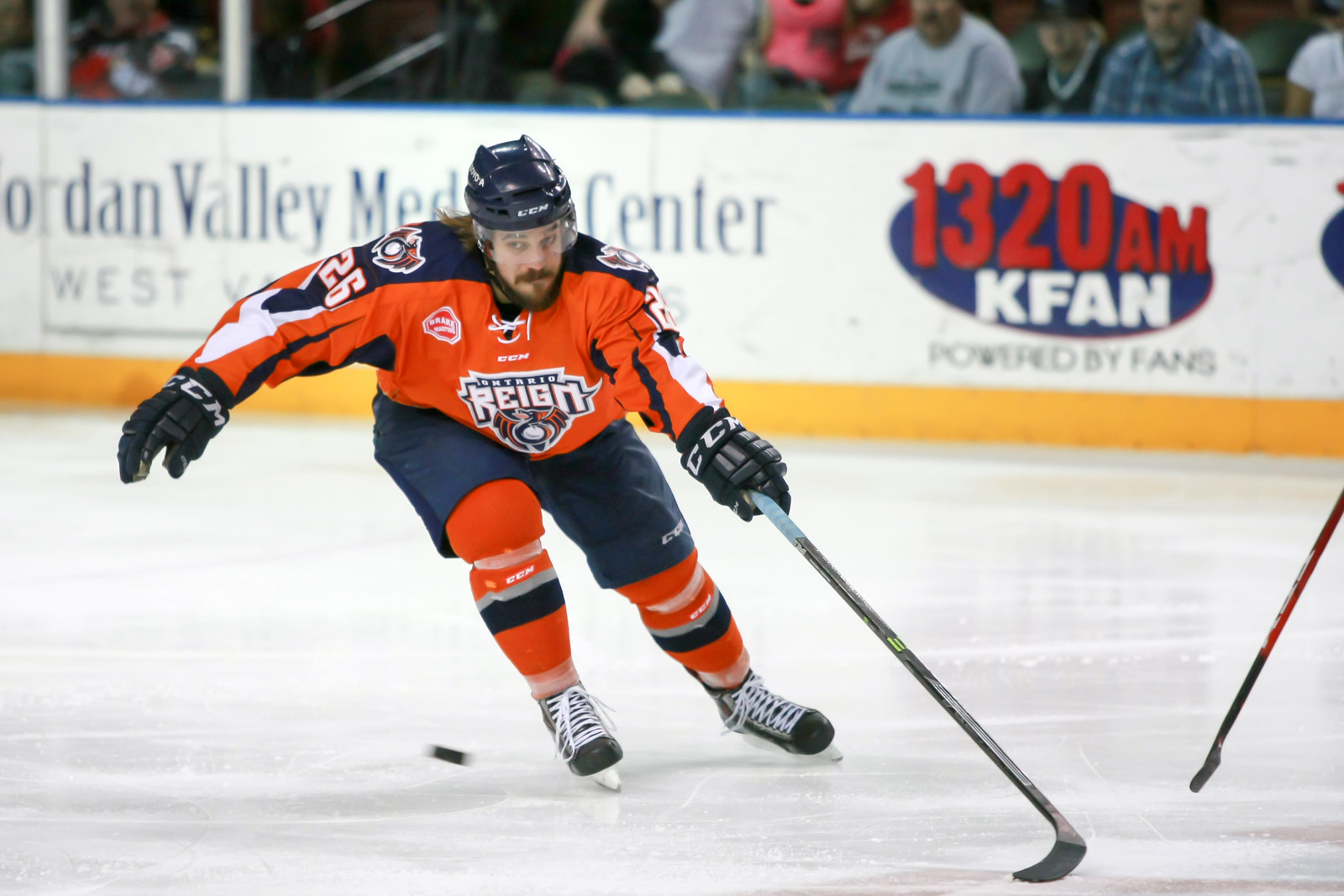The photograph captures a dynamic moment in an indoor hockey rink where a primary focus is on a middle-aged white hockey player, who appears poised to either hit or has just hit the puck. The player, adorned in a hockey uniform featuring a jersey with “Rain” on the front, sports a combination of orange, navy blue, and white colors—an orange jersey with blue sleeves and shoulders, blue knee-length shorts, and orange knee guards with blue and gray stripes. His gear includes black-lace hockey skates, heavy gloves, and a blue helmet. He also has a mustache and a beard. 

In the background, a barrier adorned with advertisements for Jordan Valley Medical Center and 1320 AM KFAN, powered by fans, separates the rink from spectators. The spectators can be seen sitting beyond the barrier, intently watching the hockey game unfold. The ice beneath glistens, and a hockey puck lies in the foreground, with the stick of another unseen player entering the frame from the right side. The scene is vibrant with the energy of the game as players vie for control of the puck.